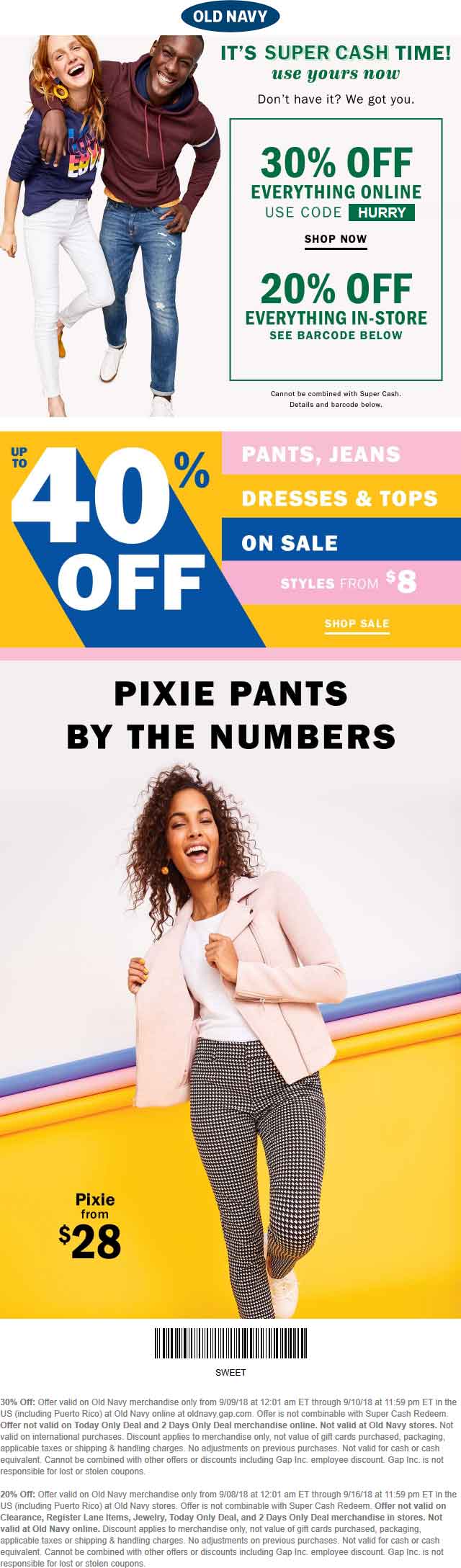Here's a cleaned-up and detailed descriptive caption for the image:

---

The advertisement, predominantly set against a white background, is visually striking with sections of bright mustard yellow, navy blue, and pink. At the very top center, there is an oval-shaped logo featuring the brand name "Old Navy" in white text against a navy blue background.

Beneath the logo, to the left, stands a woman wearing white pants and a printed tee. Beside her, a smiling man with a red top and jeans has his arm around her shoulder. Both individuals are smiling broadly; the woman is white, and the man is black.

Adjacent to them on the right-hand side, written in green, is the phrase "It's Super Cash Time. Use Yours Now." Below this text, smaller black lettering provides additional information, followed by a green-outlined square. Within this square, it states "30% off everything online" and "20% off everything in store," accompanied by further details in smaller print.

The banner below features a deep bright yellow background. On the left-hand side of the banner, "40% off" is displayed in white with a navy shadow effect. On the right-hand side, a pink bar at the top reads "Pants/Jeans," and below in the yellow section, it says "Dresses and Tops." A navy bar labeled "On Sale" follows, along with a pink bar containing text that includes a visible "$8." The final yellow bar also contains some small white text.

The lower half of the image prominently features "Pixie Pants by the Numbers." A stylish black woman with beautifully curly hair is modeling striped pants, a white top, and a pink jacket. The backdrop behind her upper body is primarily white, intersected by a diagonal line of blue, pink, and yellow from the lower left to the upper right. The section behind her legs is mustard yellow, displaying a price of "$28."

Additionally, beneath the model, there's a barcode and tiny font likely detailing terms and conditions.